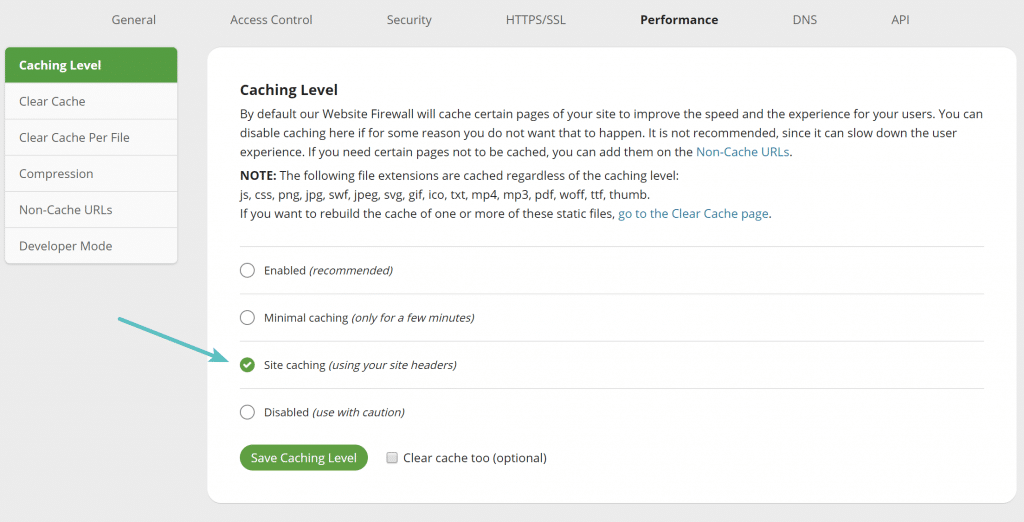In this screenshot set against a solid white background, the upper left corner features a navigation menu with the following options listed in gray text from left to right: "General," "Access Control," "Security," "HTTPS/SSL," "Performance" (highlighted in bold black), "DNS," and "API." Beneath this navigation area on the left, "Caching Level" is prominently displayed in green text.

Directly below, in white text, the options "Clear Cache," "Clear Cache per File," "Compression," "Non-Cache URLs," and "Developer Mode" are listed. To the right, under the "Caching Level" header, four options are presented, each accompanied by a small circle to indicate selection status. These options include: "Enabled," "Recommended," "Minimal Caching (Only for a Few Minutes)," and "Site Caching (Using Your Site Headers)," with the last one being checked off. The final option, "Disable (Use with Caution)," appears last in the list.